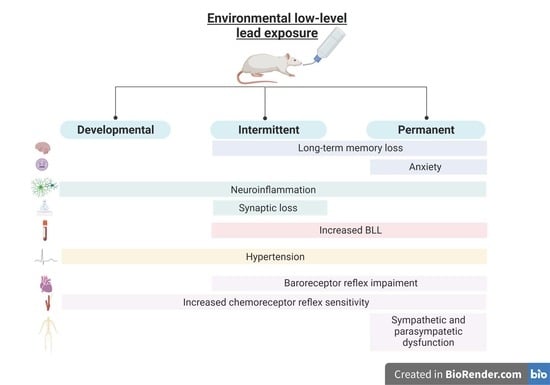The image depicts an educational chart titled "Environmental Low-Level Lead Exposure," created in BioRender.com. At the top of the chart is a contemporary illustration of a white mouse drinking from a clear water bottle. Below the title, there are three main columns labeled "Developmental," "Intermittent," and "Permanent." These columns organize a series of symptoms and factors associated with lead exposure. The chart is detailed with many labels, text, and vertically oriented images in soft colors of green, pink, and yellow, creating a modern visual appeal. It seems aimed at showing the progression and effects of lead exposure over time, starting from the point of onset. Specific symptoms are categorized within the columns: for instance, neuroinflammation is noted under all three columns, while long-term memory loss is under both intermittent and permanent, and anxiety is listed solely under permanent. This intricate diagram, featuring rows of symptoms such as synaptic loss, hypertension development, and increased chemoreceptor reflex sensitivity, appears designed for those with a scientific background, explaining various stages and impacts of low-level lead exposure.